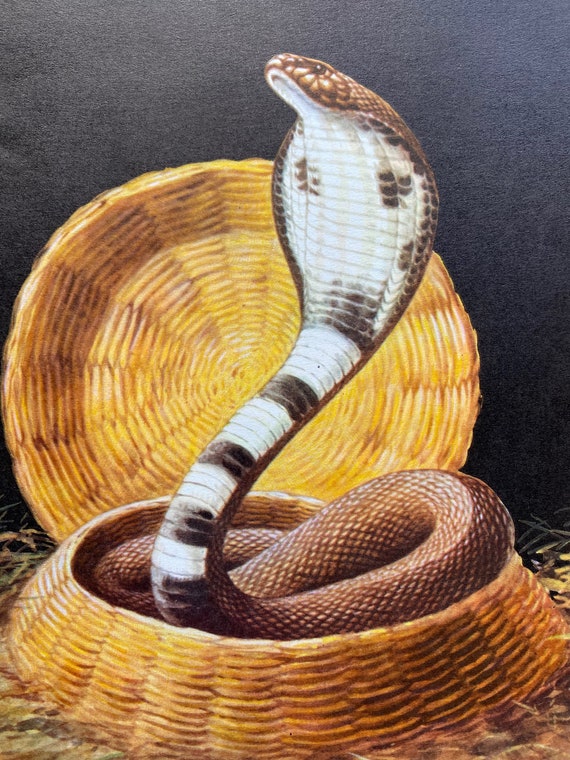This image depicts a captivating painting of a cobra, dramatically coiled within a large, straw basket. The cobra's body, adorned with a distinct brown diamond pattern on top and white stripes underneath, ascends gracefully from the center of the basket, with its head slightly tilted towards the left. Its left eye gleams, conveying a sense of alertness, while its mouth remains closed, suggesting it might be charmed. The intricately designed basket, rendered in shades of brownish-yellow, rests atop a patch of straw or grass, adding a natural, rustic element to the scene. The basket's lid leans against a stark black wall in the background, drawing further attention to the ornate details of the basket and the snake. The entire composition, with its old-school aesthetic, evokes imagery reminiscent of illustrations from a vintage children's book.